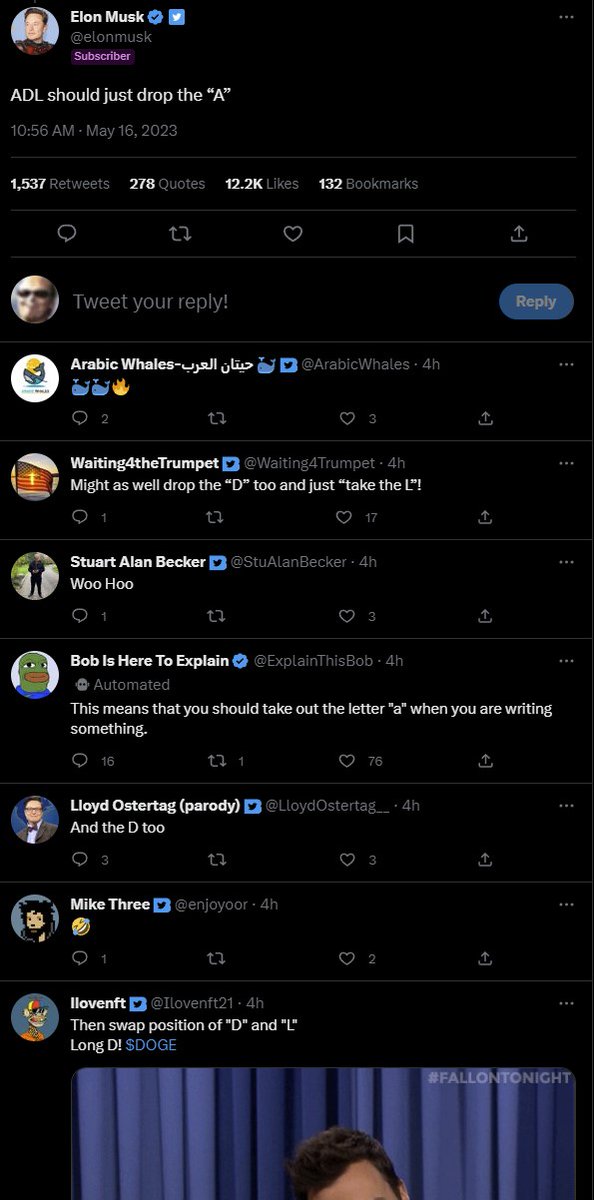In this Twitter post, located in the top left corner of the image, Elon Musk's profile is prominently featured. His profile picture, depicting Elon Musk himself, is positioned next to his verified handle "@elonmusk" and marked with a subscription tag "Subscriber" written in purple. His tweet reads, "ADL should just drop the 'A'", and it's timestamped "10:56 a.m. May 16th, 2023". This tweet has garnered significant engagement, with 1,537 retweets, 278 quotes, 12.2K likes, and 132 bookmarks.

Beneath this, the interface shows the standard interaction icons: a chat bubble for replies, a retweet icon, a heart for likes, a bookmark symbol, and an upload button. Below these icons, there is a section inviting users to "Tweet your reply", accompanied by a user's face next to the prompt. To the right of this prompt is a blue button labeled "Reply" in white text.

Further down, the image shows a series of seven replies to Elon Musk’s tweet, filled with various user comments. At the bottom of the image, there is a partial view of Jimmy Fallon, recognizable by the backdrop of his stage, paired with the hashtag "#FallonTonight".